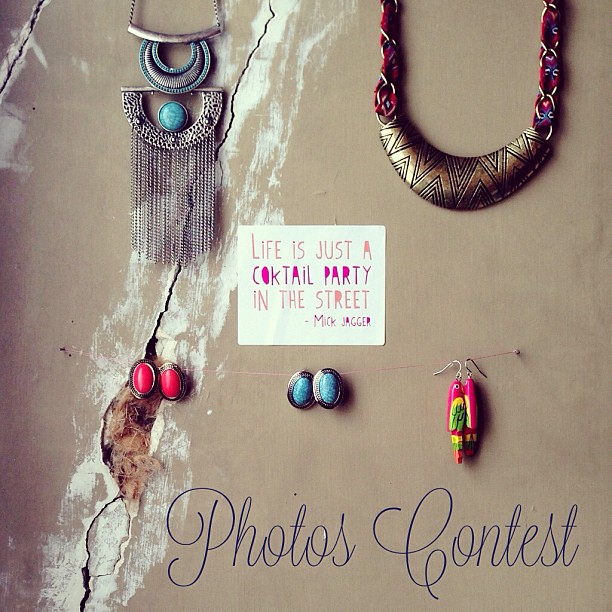The image is a color photograph of various jewelry pieces, set against a cracked and streaked beige concrete or plaster background, giving it a rugged texture. In the upper left corner, there's a pendant necklace with silver chains adorned with turquoise stones. To the upper right, there's a striking gold medallion necklace featuring multicolored red and blue threads, giving it a tribal aesthetic. Centrally placed is a white square featuring a quote in decorative peach and pink font that reads, "Life is just a cocktail party in the street," attributed to Mick Jagger. Below this quote, three sets of earrings are arranged in a row: on the left, earrings with red stones; in the middle, earrings with turquoise stones; and on the right, parrot-shaped earrings with pink, yellow, and green colors. In the bottom right corner of the image, blue text in a cursive, handwriting-like font proclaims "Photos Contest."